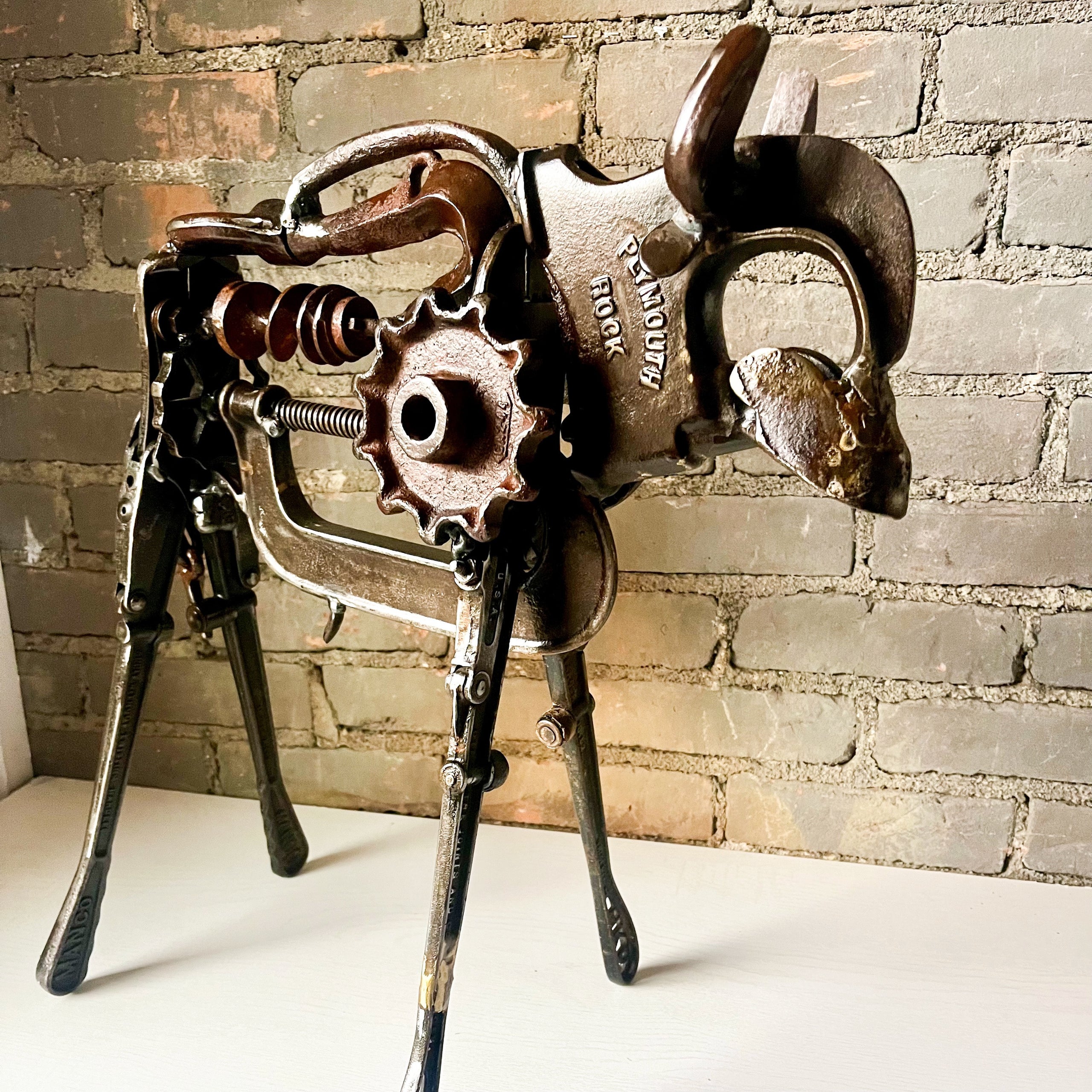The image captures an intricate and artistic sculpture of a bull, crafted from recycled metal machinery parts and tools. The bull stands erect on a plain white table, set against an aged brick wall with crumbling mortar, hinting at warm red and grey tones. This imaginative pastiche is composed of various gears, iron tools, and welded metal items, giving it a dark, metallic sheen. The sculpture boasts four spindly legs and is adorned with two prominent horns on its head. Notably, the bull's neck features the text "Plymouth Rock" stamped into the metal. The detailed construction includes elements such as a gear in the shoulder area, adding to its mechanical charm. This unique artwork is both a testament to creative recycling and meticulous craftsmanship.